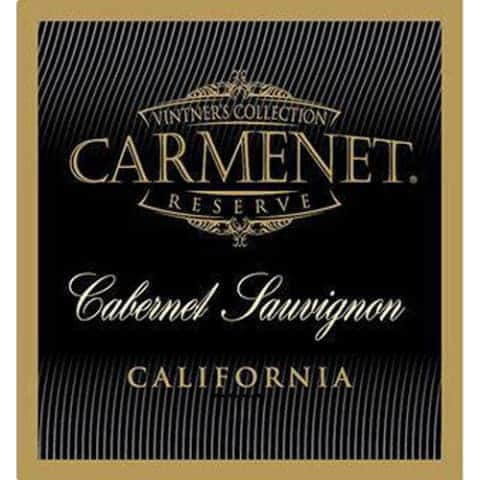The image shows an elegant and sophisticated label set against a stylish black background, decorated with vertical gold stripes at the top and bottom that gradually fade into the background. Encasing the label is a plain gold border that adds to its refined aesthetic. Prominently featured in the center, the text displays "Vintner's Collection" in gold, followed by "Reserve" and "Cabernet Sauvignon," with "California" also inscribed in gold at the bottom. The positioning of the text is well-arranged, lending the label an overall balanced and polished appearance. The use of black, gold, brown, gray, and white colors suggests a high-end, upscale design, reminiscent of an advertisement or label for a premium wine, perhaps intended to be seen in a fancy restaurant or on a luxury product website.